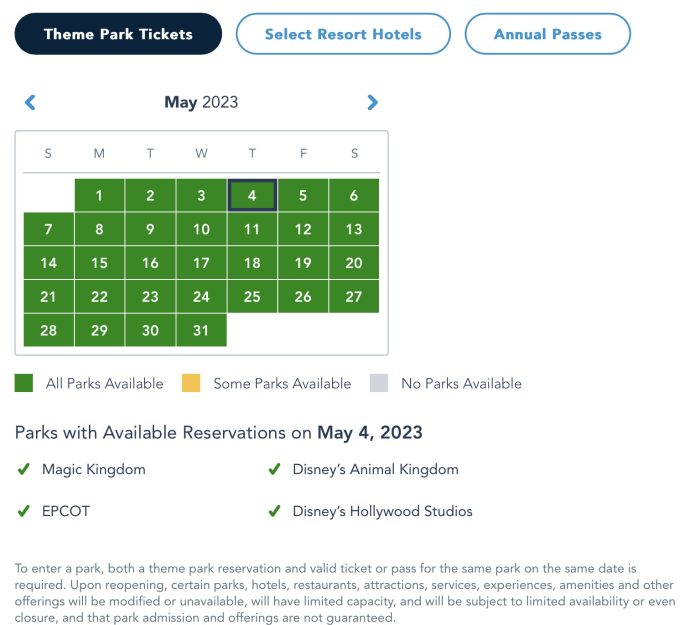This image depicts the Disney booking page interface. The background is primarily white, and at the top of the page, there are three clickable buttons designed as bubbles. These buttons offer options for "Theme Park Tickets," "Select Resort Hotels," and "Annual Passes."

Directly beneath these buttons lies a calendar interface for managing bookings. The calendar display features navigational arrows on either side at the top, which allow users to scroll through different months. Centrally located at the top of the calendar section, "May 2023" is prominently displayed, indicating the current month being viewed.

Within the calendar grid, each day of the week is represented by tiles. For May 2023, the tiles are predominantly green, symbolizing availability. Below the calendar, a key is illustrated to help users decipher the tile color coding: green tiles indicate all parks are available, yellow tiles denote some parks are available, and gray tiles signify no parks are available.

Continuing down the page, there's a section highlighting "Parks with available reservations on May 4th, 2023." Listed here are Magic Kingdom, Epcot, Disney's Animal Kingdom, and Disney's Hollywood Studios. Each park name is accompanied by a green checkmark on the left side, signifying that all four parks have open and available reservations for that specific date.